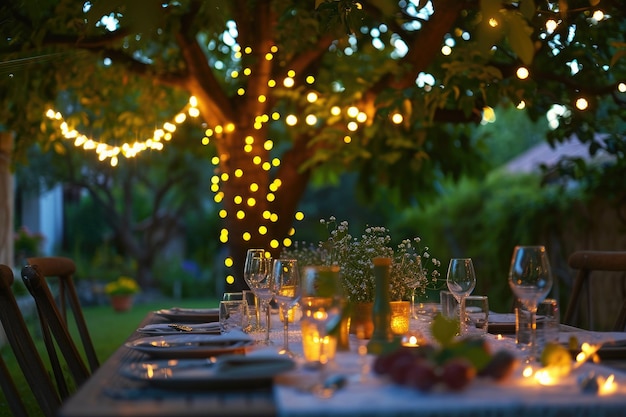This photograph captures a beautifully arranged dinner table set for an alfresco meal. Dominating the background is a tall tree adorned with strings of twinkling white lights wrapped around its branches, while circular yellow lights encircle its trunk, casting a warm glow. To the right, a brown wooden fence is partially obscured by cascading greenery, adding a natural touch, while a garden brimming with blue and yellow flowers enhances the picturesque scene. The dinner table itself is meticulously set with elegant plates and clear wine glasses, featuring small yellow votive candles scattered across its surface. A table runner down the center boasts a charming display of fresh fruit and greenery. Surrounding the table are wooden indoor-style chairs, contributing to the inviting ambiance. The photograph, taken from a low angle at the end of the table, effectively draws the viewer's eye down the length of this enchanting setup, making one feel as though they are about to join the gathering.